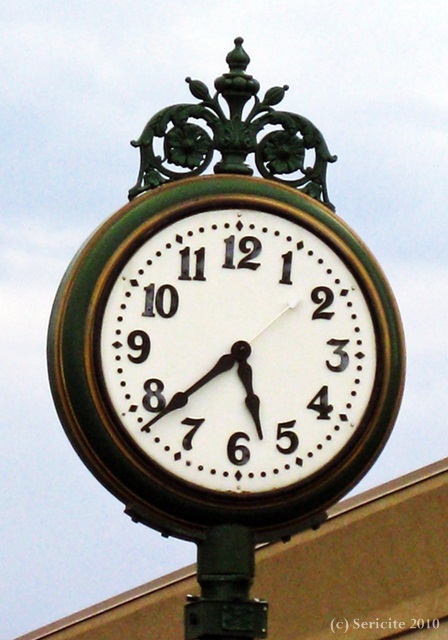This photograph captures a striking outdoor timepiece mounted on a decorative lighting pole, resembling the classic city clocks often found in urban squares or theme parks like Disneyland. The clock, crafted from a green metal, features large, prominent numbers from 1 to 12, interspersed with four smaller dots between each hour, enhancing its ornate design. Adding to its elegance, the outer rim of the clock is adorned with gold trim, which, though seemingly worn in places, appears to be an intentional design choice. Above the face, an intricate floral carriage with two small flowers adds a touch of charm. The sturdy pole supporting the clock showcases a complementary green and black pattern, blending both functionality and style. In the bottom right corner of the image, the logo "Ceracite 2010" signifies the photographer's copyright.